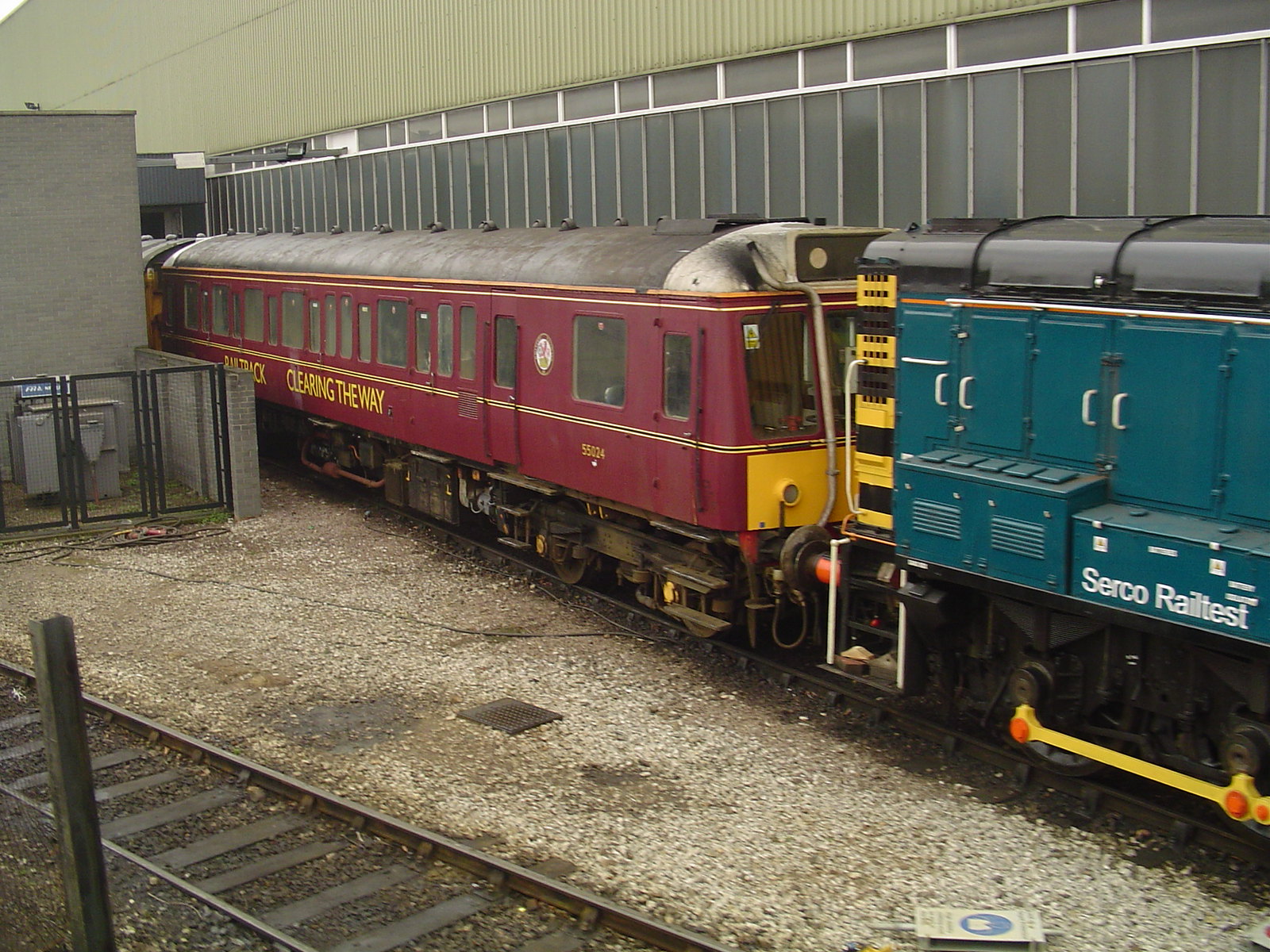The photograph captures a scene of two connected railroad cars in a rail yard, emerging from a man-made tunnel. The blue front car has the text "Sergo Rail Test" printed on it, while the red car with yellow trim behind it carries the text "Clearing the Way." This setup suggests these might be specialty cars designed for clearing tracks of snow or debris. To the rear, a large fence and what appears to be a train depot or a gray building provide a backdrop. Other details in the image include an empty parallel track in the foreground, dirt and gravel between the tracks, and a possible electrical equipment building in the upper left corner. The trains themselves are in good condition, with visible surroundings that include a deep gray wall and a white barrier atop it, with additional structures nearby.